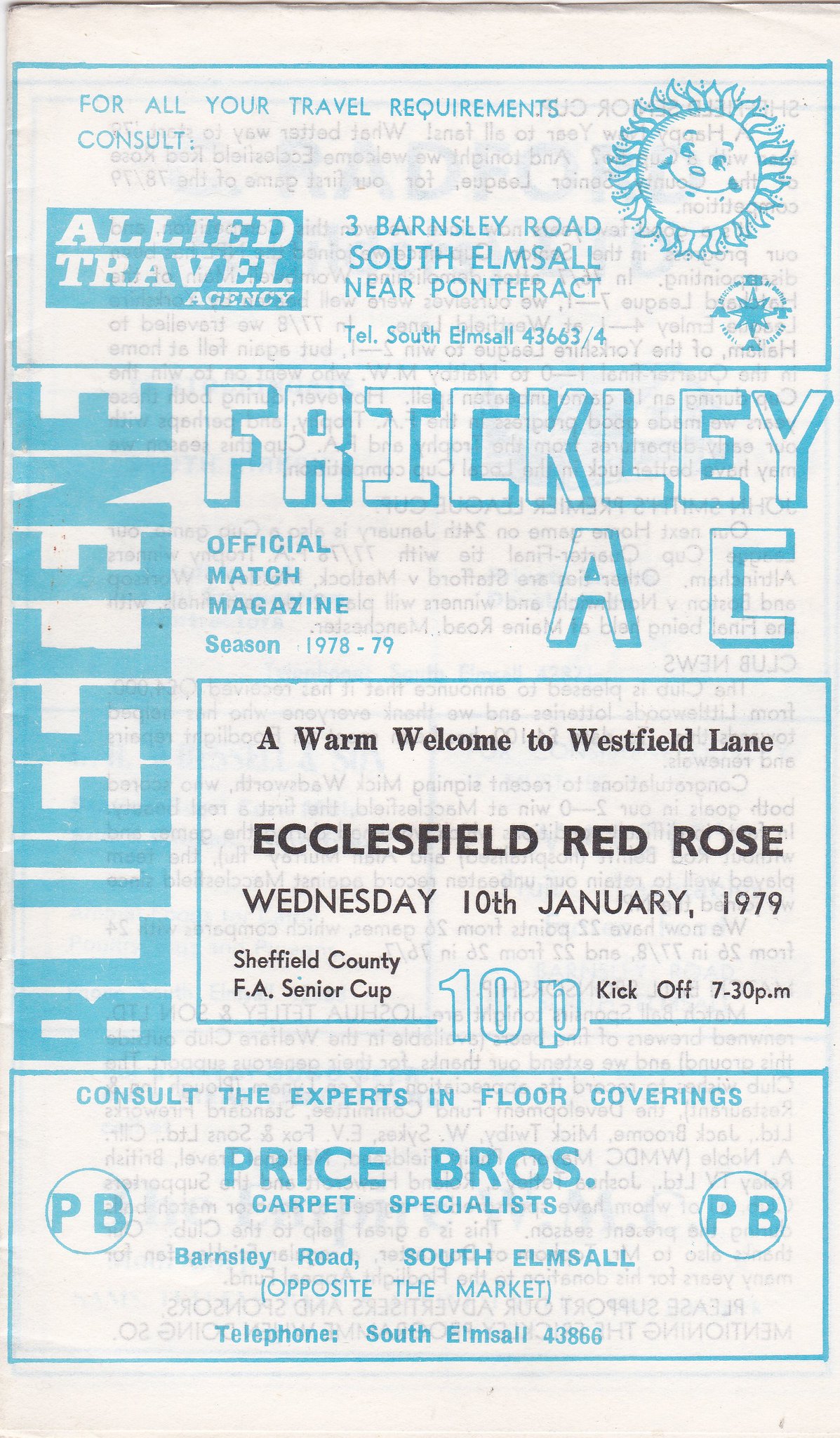This is the cover of an official match program booklet from Frickley A.C. for their 1978-1979 soccer season. The program, designed on very thin, off-white paper, features a blue-outlined rectangular header at the top, which advertises the Allied Travel Agency with their address (3 Barnsley Road, South Elmsall near Pontefract) and phone number (South Elmsall 43-663-4), along with a small cartoon sun in the upper right corner and a compass rose marked A-B-A-T. Beneath this, in blue block letters, it states "Frickley A.C. Official Match Magazine Season 1978-79." Further details include a warm welcome to Westfield Lane for a match against Ecclesfield Red Rose on Wednesday, January 10th, 1979, part of the Sheffield County F.A. Senior Cup, with a kickoff time of 7.30 p.m., and an entry price of 10p. Along the spine of the page, the text "Blue Scene" can be seen, and below the match details, there is an advertisement promoting Price Bros, carpet specialists, with their location and contact information.